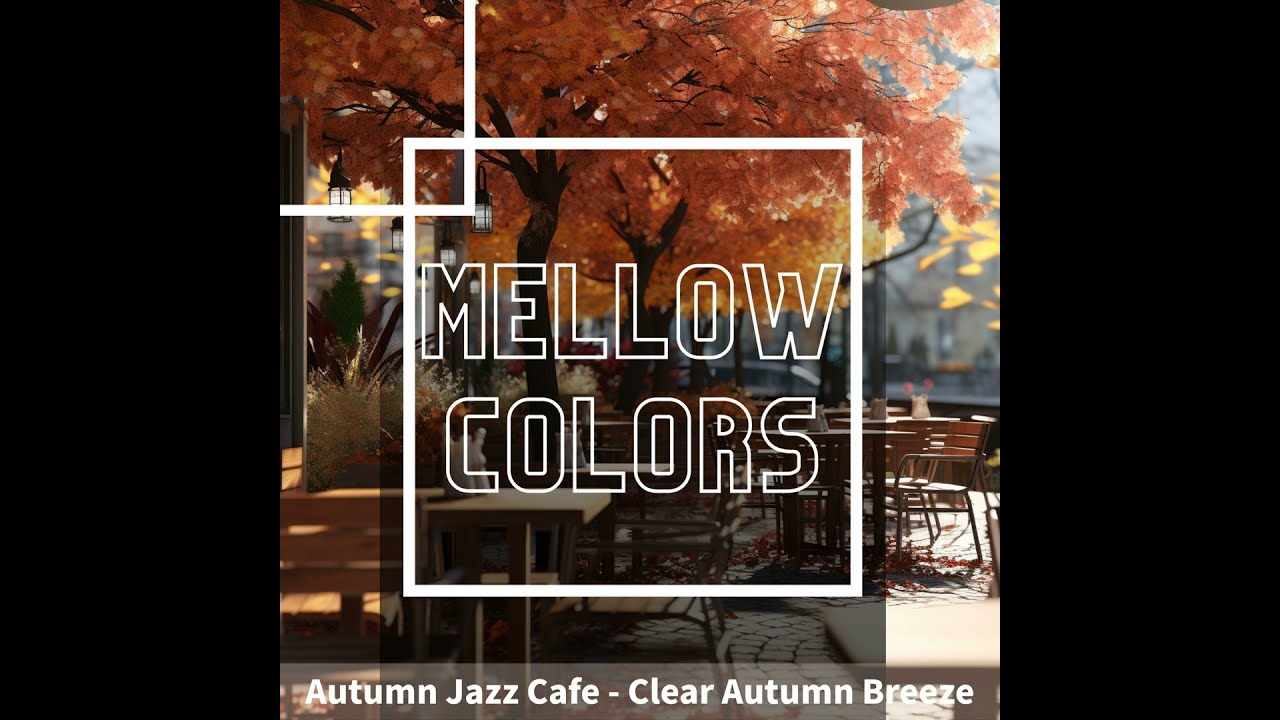This image, likely an advertisement for an autumn-themed establishment, depicts a tranquil outdoor setting at a sidewalk cafe. Central in the scene is a vibrant autumn tree with pink, yellow, and red leaves, standing amidst the cafe’s brown, cobblestone-paved area. The cafe's setup includes wooden tables and metal-framed chairs, arranged seemingly in an inviting manner, although currently unoccupied. The trees have striking black trunks, accentuated by the colorful foliage. In the upper left, several black and white lanterns hang from posts and trees. Surrounding this image are black rectangles on the left and right, enhancing the central focus. Overlaid on the photograph, within a white square, is the text "Mellow Colors." Below, a gray stripe at the bottom bears the words "Autumn Jazz Cafe - Clear Autumn Breeze," encapsulating a serene, jazz-infused autumn ambiance.